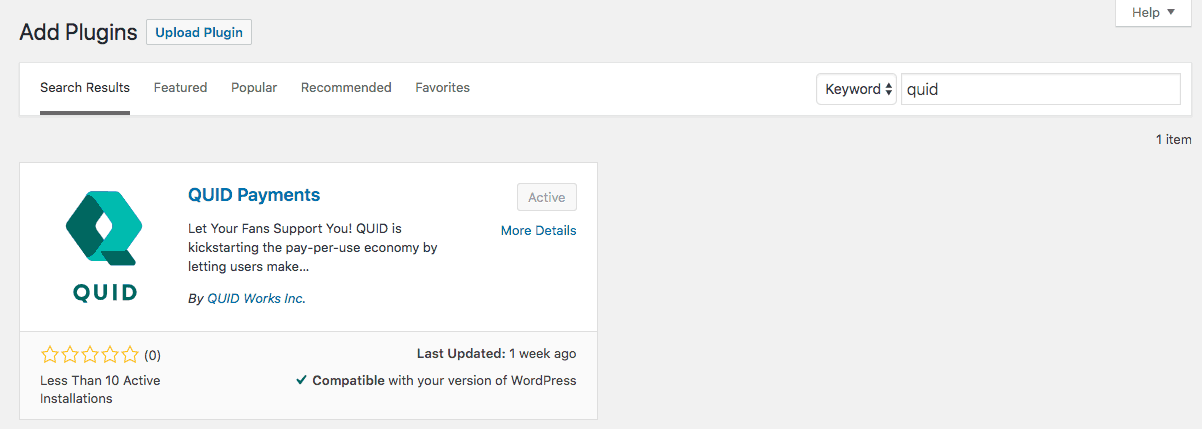The image displays a horizontal, left-to-right interface typical of a computer smart device. The background is a sleek gray tone. In the upper left corner, bold black text reads “Add Plugins.” Below this, a small rectangular button in gray with blue letters states “Upload Plugin.” On the opposite corner at the top right, a white “Help” button featuring a downward arrow indicates more options.

Beneath the "Add Plugins" title, a long, thin rectangular white strip is visible with various selectable options. The option “Search results” is highlighted with a black underline, followed by “Featured,” “Popular,” “Recommended,” and “Favorites.” To the right of these tabs, there is a search field labeled “Keyword” with the text “quid” currently entered. Directly below this search field on the right, it shows “1 item found.”

On the left, underneath the search options, a prominent white box with a gray lower section appears. Inside the white section, there is a blue icon for Quid. Next to this, the text reads “Quid Payments: Let your fans support you. Quid is kick-starting the pay-per-use economy by letting users make…” The plugin summary is attributed to “Quid Works Inc.”

To the right of this text, there is an active button labeled “More Details.” In the gray lower portion, there is a star rating system with no stars filled in, indicating “0 reviews.” Additional information mentions, “Less than 10 active installations, last updated one week ago, and compatibility with your version of WordPress.”